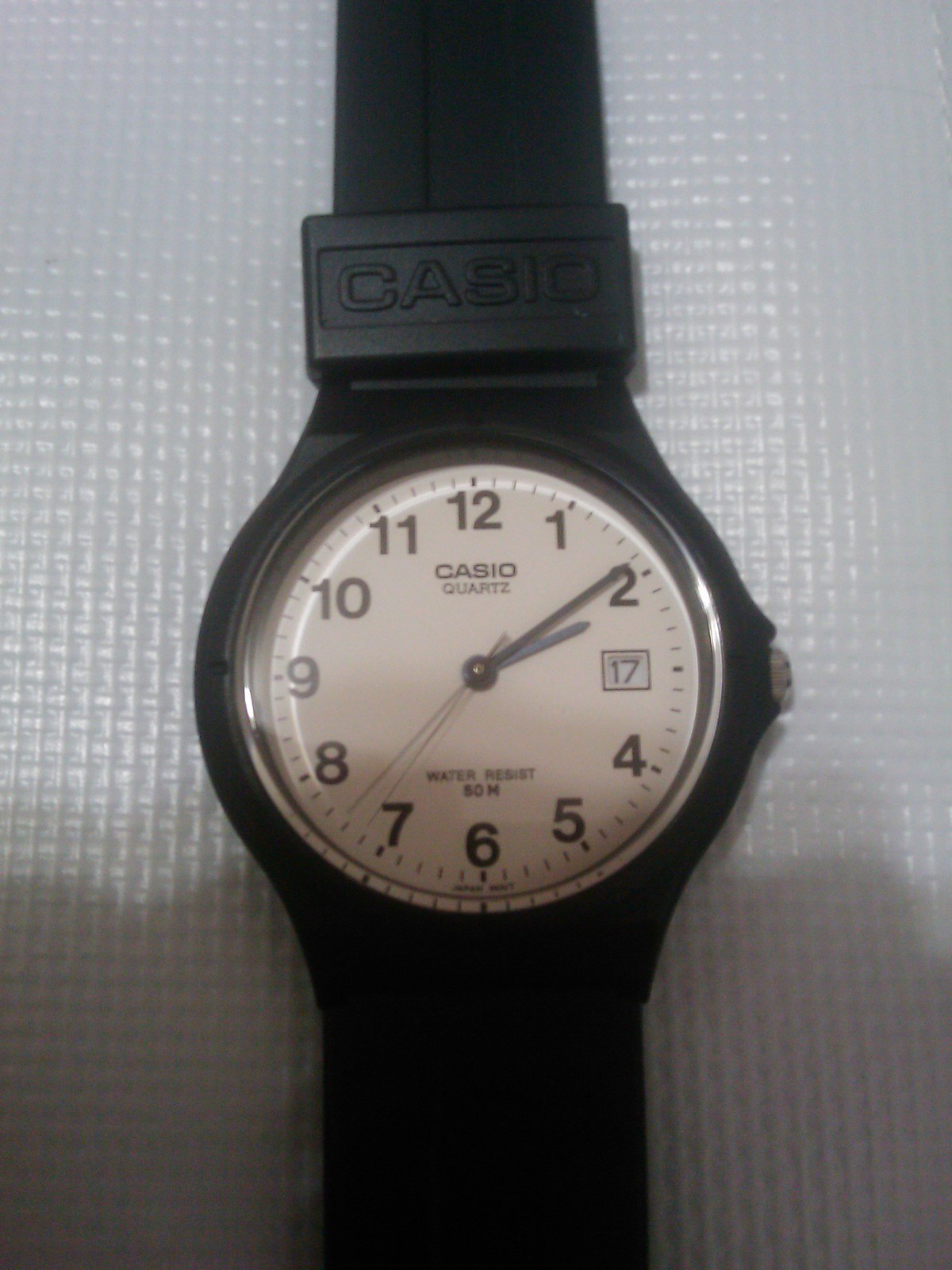This image, captured in a vertical orientation likely with a phone camera, depicts a black Casio Quartz wristwatch lying flat on a white, textured, somewhat plasticky surface. The watch features a circular analog display with a white face and black numbers denoting hours 1 through 12, along with smaller lines for seconds between each number. The hours are marked by black text, and the time is shown with two main black dial hands for the hour and minute, along with a very thin needle-like hand for seconds. Notably, where the number 3 would typically be, there is a small square window displaying the number 17, likely indicating the date. The wristband and frame of the watch appear to be made of a rubbery plastic material, reminiscent of a sports watch, although it is not digital. The photo features a shadow in the bottom quarter, presumably from the photographer, adding a subtle dynamic element to the otherwise static scene. The time displayed on the watch reads approximately 2:09.